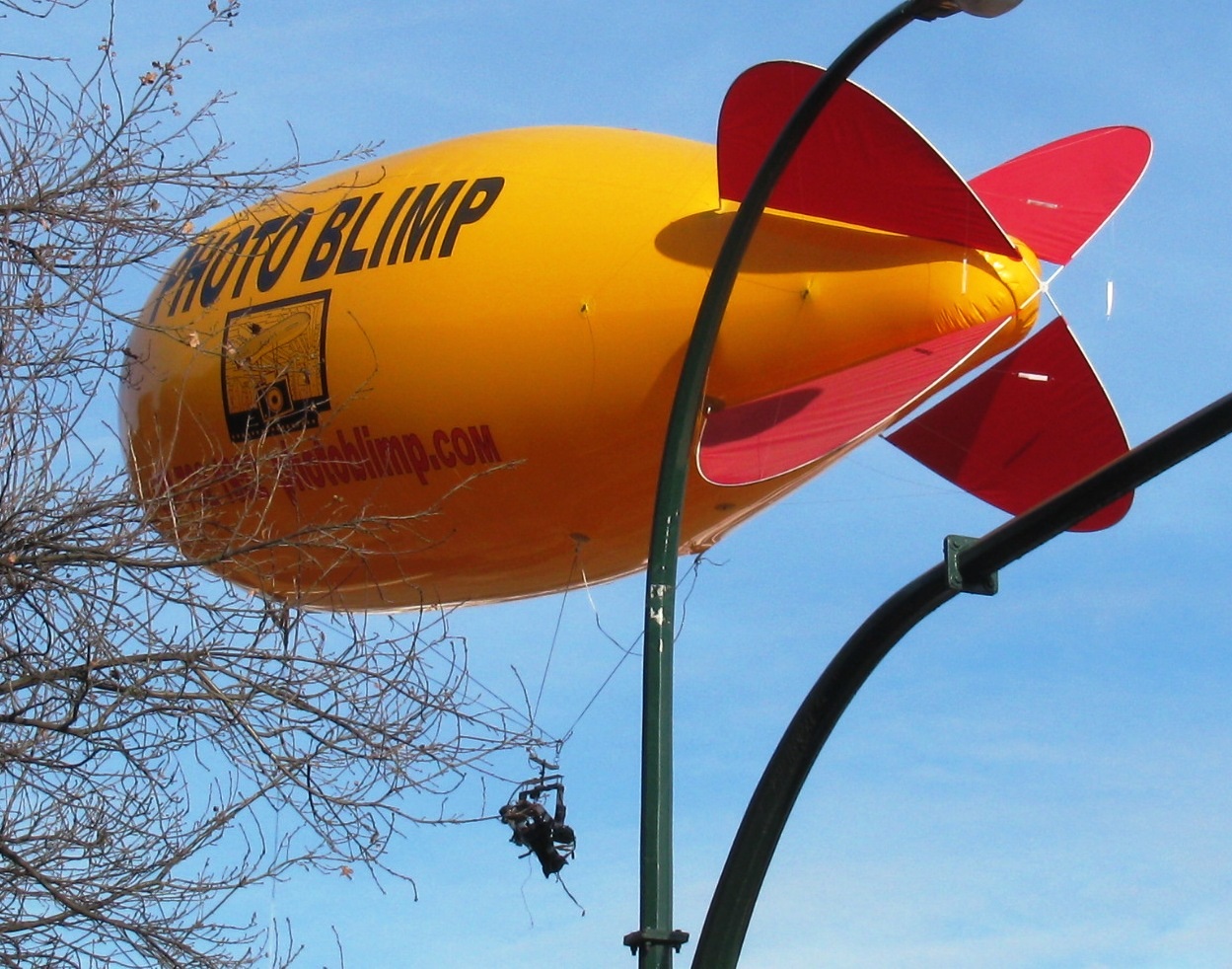In this image, a bright yellow blimp, labeled "photo blimp" in bold black letters, floats in a clear, light blue sky. The blimp, which has red markings including a propeller at its rear, prominently features the website "photoblimp.com" in red letters on its side, although part of the text is obscured by the bare branches of a nearby tree. The blimp also displays a square picture and seems to be pointing to the left. Suspended beneath the blimp by tethers is a black camera apparatus held by a U-shaped metal bar. The bottom part of the image has the curved steel arms of what appears to be a street lamp, partially visible and casting a slight shadow on the scene. The overall composition is horizontally oriented, emphasizing both the blimp and its surroundings.